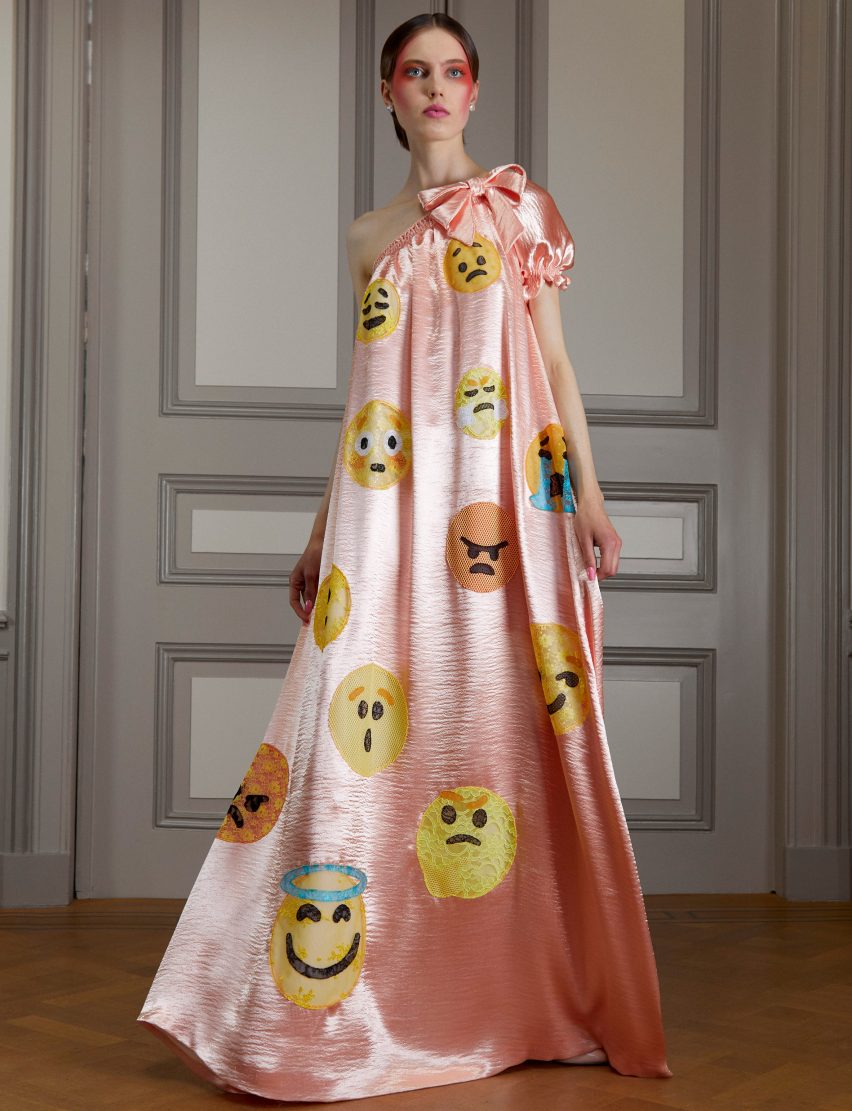In the image, a Caucasian woman with her dark brown hair tied back into a tight bun models an off-the-shoulder, shimmering metallic pink dress that cascades down to the floor. The dress is adorned with various stitched-on emojis, including angry, surprised, thinking, blushing, crying, angelic, and frowning faces. The woman has white skin accentuated by heavy makeup, featuring dramatic red mascara and under-eye paint extending down to her cheeks, along with lipstick and pearl-like earrings. Her right shoulder is bare, further highlighting the elegance of the garment. She stands in front of large beige-gray double doors, with a brown to tan-colored floor beneath her, possibly in a grand mansion setting. A pink bow accessory adorns the top corner of the dress, completing her striking appearance.